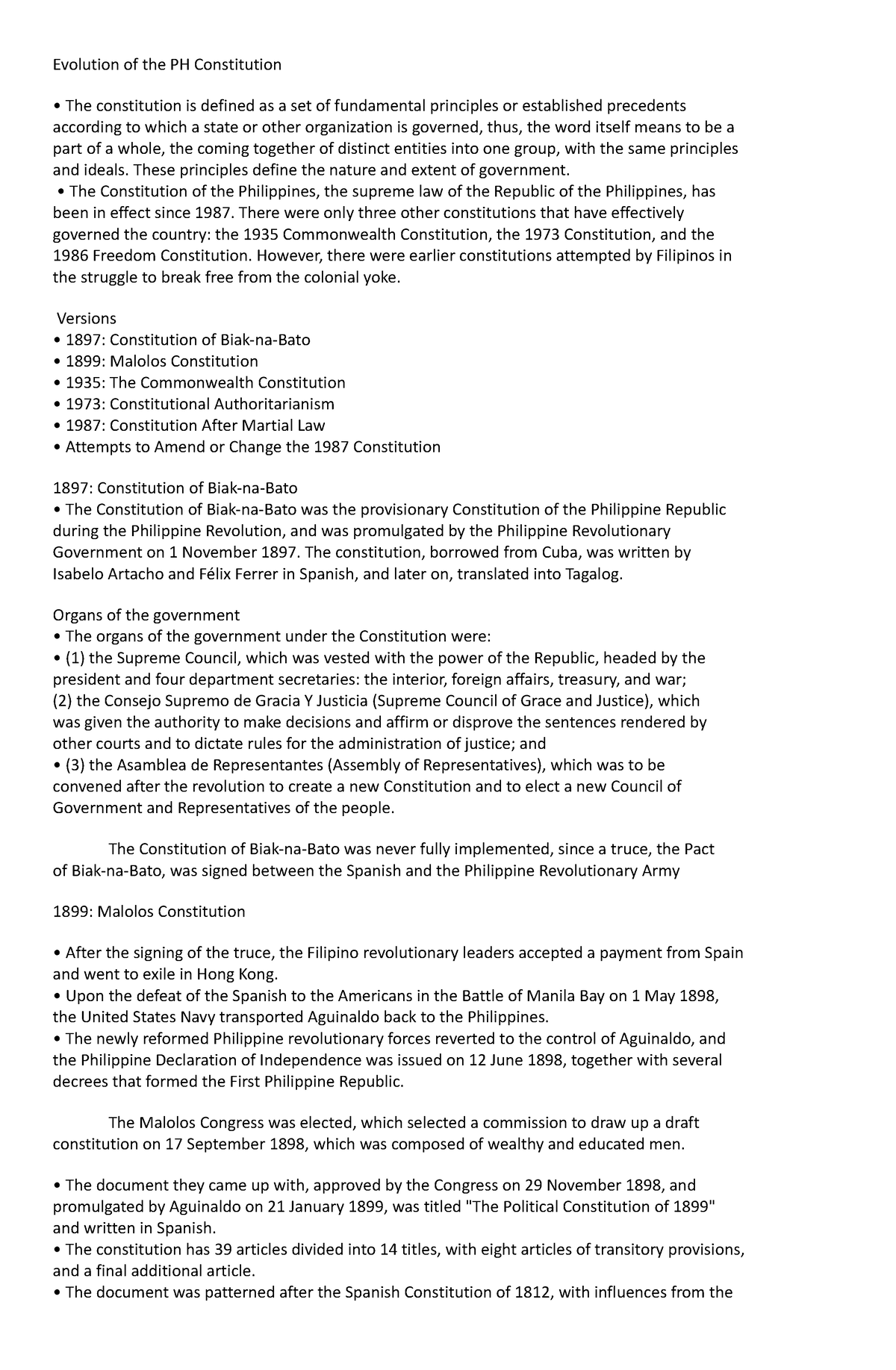This image showcases a detailed, chronological evolution of the Philippine Constitution against a white background. The timeline begins with the 1897 Constitution of Biak-na-Bato, highlighting its historical context and significance in the struggle for independence. It then features the 1899 Malolos Constitution, the first republican constitution in Asia. The 1935 Commonwealth Constitution is next, reflecting the transitional governance under U.S. sovereignty. Moving forward, the image describes the 1973 Constitution implemented under the Marcos regime, known for its authoritarian amendments. The timeline leads to the 1987 Constitution established post-martial law, which aimed to restore democracy and civil liberties. Alongside, it mentions several attempts to amend this version. The narrative concludes noting that the 1897 Constitution of Biak-na-Bato was never fully implemented due to the truce signed in the Pact of Biak-na-Bato between the Spanish and the Philippine Revolutionary Army.